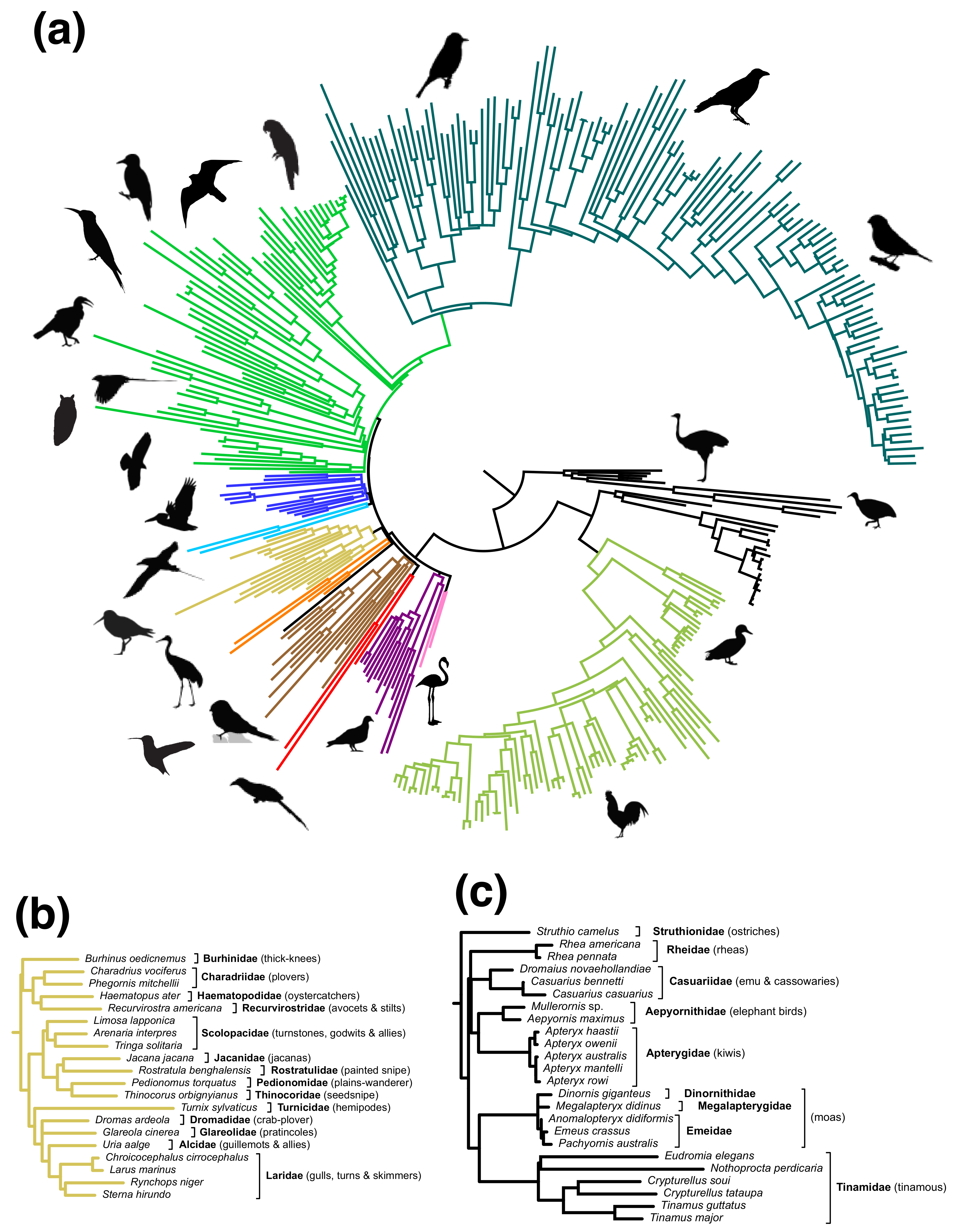The infographic presents a detailed, spiral-shaped diagram illustrating the evolutionary connections between various bird families. This colorful flowchart, labeled Part A, features multiple branches with different hues, representing diverse bird genera and species. Black silhouettes of birds, including ostrich, emu, wren, robin, eagle, sparrow, flamingo, rooster, duck, hummingbird, and chicken, adorn the chart's white background. The diagram is complex and resembles a family tree or flowchart, with numerous intersecting lines depicting the intricate relationships within the avian world. Parts B and C, located beneath the spiral, contain explanations in Latin and English, although the text is too small to read clearly. These sections list the scientific names of bird groups, including many notable species like thick-knees, plovers, oyster catchers, avocets and stilts, turnstones, godwits and allies, among others.